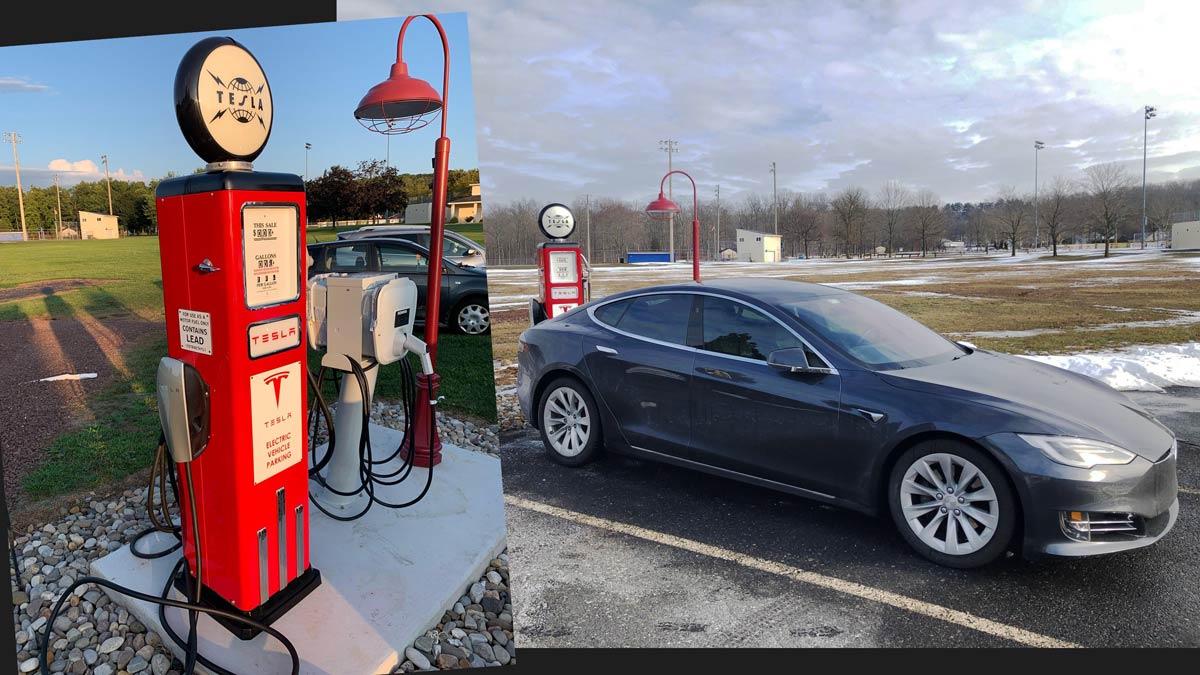This composite image features two photos side-by-side, highlighting a modern twist on vintage aesthetics. On the left, there is a Tesla-branded electric vehicle (EV) charging station designed to mimic a 1920s to 1940s gas pump. The red, tall stand sports a round white top with blue lettering spelling "Tesla." The pump features analog-style dials and numbers in the center, and an electric pump handle is notably attached to the side. Adjacent stands an old-fashioned lamppost, contributing to the nostalgic look. On the right, a four-door black Tesla sedan is parked in front of this vintage-inspired charging station. The surroundings show a grassy park-like area with some trees and hints of snow, adding to the serene outdoor setting.